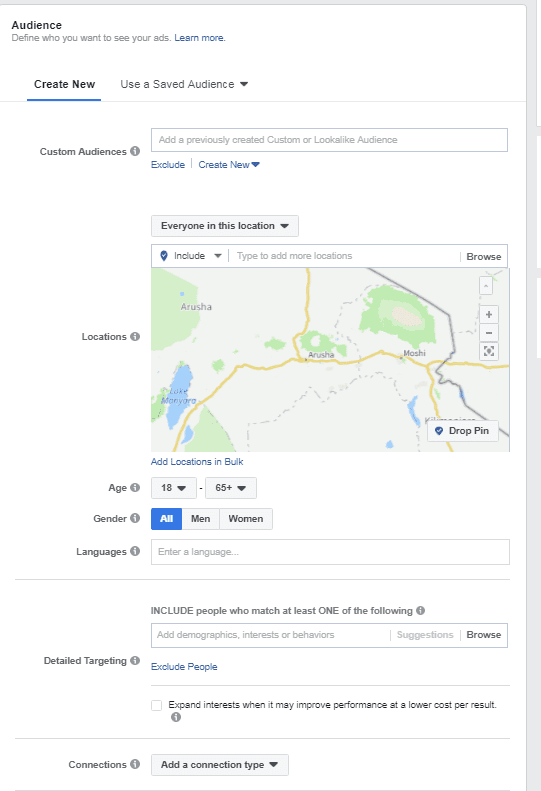The image displays a webpage with a clean, white background. At the top, in bold black text, the heading reads "audience," followed by a subheading in lighter gray text that says "define who you want to see your apps." To the right of this subheading is a "learn more" link in blue text.

Further down, another bold heading says "create new," underlined with a blue line, adjacent to the option "use a saved audience" which includes a drop-down menu. Below, a section labeled "custom audiences" features a search bar with the instruction "add a previously created custom or lookalike audience." 

Another drop-down menu, labeled "exclude," in blue text follows beneath. A small rectangular section next displays the text "everyone in this location" alongside a drop-down menu. Directly below, a banner includes the text "include" in a drop-down menu and an option to "type to add more locations and browse."

To the side, another label reads "locations," next to a square box showing a map. Underneath this map section, a blue text link says "add locations in bulk." 

Further down, demographic selections show age range options from "18 to 65+," gender options of "all," "men," and "women" (with "all" selected), and a text field for "languages" labeled "enter a language." 

A detailed targeting section includes instructions to "include people who match at least one of the following," with options to "add demographics, interests, or behaviors," alongside links for "suggestions," "browse," and "detail targeting." Also provided is an "exclude people" option in blue text.

At the very bottom, a square section includes the option to "expand interest when it may improve performance at a lower cost per result." Finally, there is a "connections" section with a prompt to "add a connection type" via a drop-down menu.